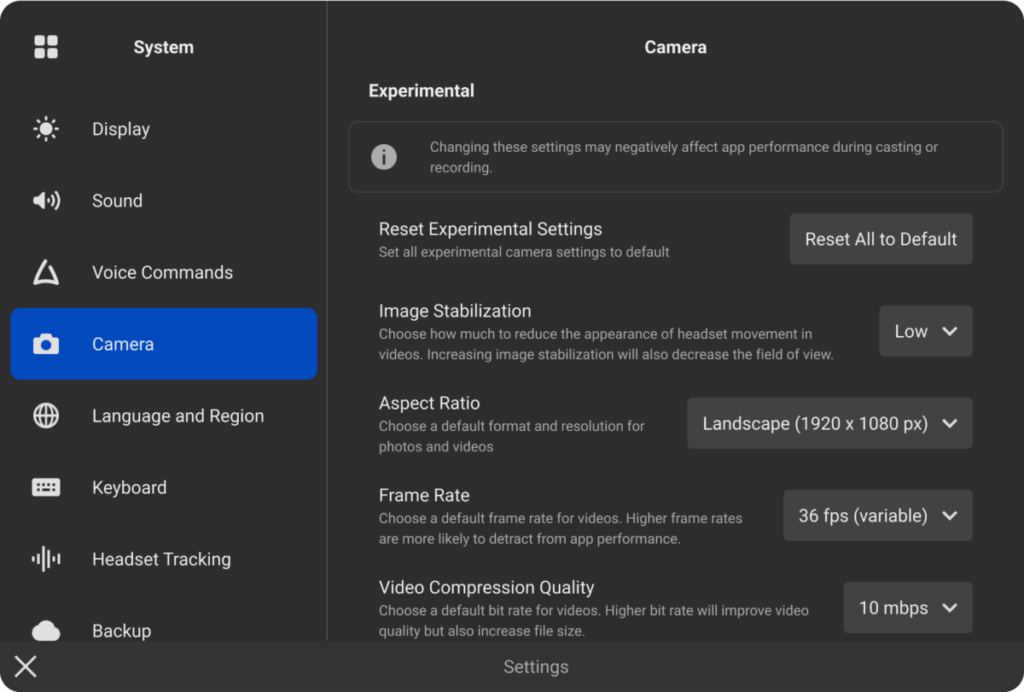The image depicts a system settings page with a black background and white text. The left section occupies about one-quarter of the screen and lists various icons and corresponding settings categories. At the top of this section, the word "System" is displayed prominently. Below it, a series of icons with text labels include:

- A brightness icon followed by the text "Display."
- A sound icon followed by the text "Sound."
- A triangle icon followed by the text "Voice Commands."
- A camera icon followed by the text "Camera," which is highlighted in blue, indicating the current selection.
- A globe icon followed by the text "Language and Region."
- A keyboard icon followed by the text "Keyboard."
- Vertical lines icon followed by the text "Headset Tracking."
- A cloud icon followed by the text "Backup."
- An exit icon at the bottom.

To the right, taking up three-quarters of the page, are detailed settings for the "Camera" section. In the center, the word "Camera" appears with the subheading "Experimental" below it. An information icon is present with a warning message: "Changing these settings may negatively affect app performance during casting or recording."

Beneath the warning, there are various settings options:

- "Reset Experimental Settings" with a button labeled "Reset All to Default."
- "Image Stabilization" with a dropdown box set to "Low."
- "Aspect Ratio" with a dropdown showing "Landscape, 1920 x 1080 pixels."
- "Frame Rate" set to "36 FPS Variable" with a dropdown arrow.
- "Wide Compression Quality" with a dropdown showing "10 Mbps."

At the bottom of this section is the word "Settings" enclosed in a border.